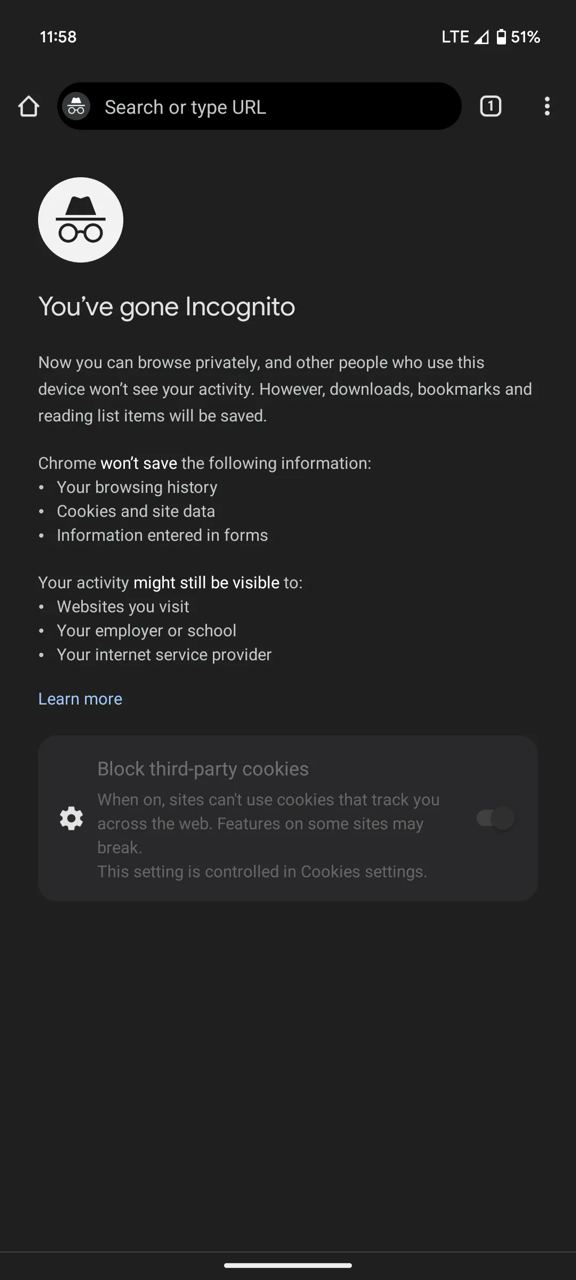This screenshot displays a mobile phone screen showcasing the Google Chrome Incognito mode. 

At the top of the screen, the status bar features a gray background. In the upper left corner, "11:58" is prominently displayed in white font, indicating the current time. In the upper right corner, the signal status shows "LTE" with half the mobile signal bars filled, next to a battery icon indicating a 51% charge.

Just below the status bar lies the Chrome Incognito interface. The top portion of the screen contains a black search field with white text that reads "Search or type URL." To the left of the search field is the incognito mode icon—a gray circle with a white hat and glasses, representing private browsing. On the right side of the search field is a small white square displaying the number "1".

Dominating the central portion of the screen is a larger incognito mode icon, featuring a white circle with a black fedora and black glasses. Below this icon, white text announces, "You've gone incognito." The text below further elaborates: "Now you can browse privately, and other people who use this device won’t see your activity. However, downloads, bookmarks, and reading list items will be saved." 

The overall theme of the image highlights the privacy features of Chrome's Incognito mode on a mobile device, marked by a minimalist design and grayscale color scheme.